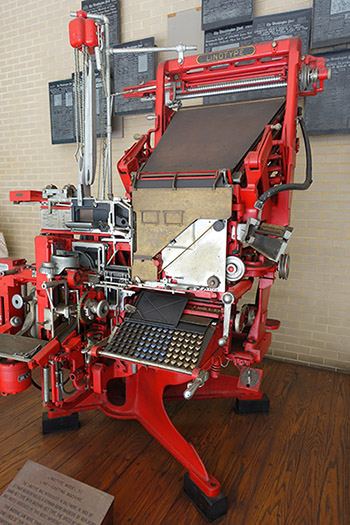The photograph depicts a large, complex red and black linotype machine situated in an interior space, likely used for producing newspapers. This imposing mechanical device, standing approximately 6 to 7 feet tall and about 4 feet wide, dominates the scene, though part of it is cut off on the left side of the image. The machine features various components including a typewriter-like keyboard at the front, a conveyor belt and rollers at the top, and numerous silver tubes and pipes suggesting a hydraulic system. Handles on the front indicate adjustable settings. The linotype machine stands on a dark hardwood floor, and the background consists of beige-white brick walls adorned with grey plaques and large black sheets with white writing, likely newspaper negatives. A brass plaque at the top of the machine explicitly identifies it as a linotype, affirming its historical use in newspaper production.